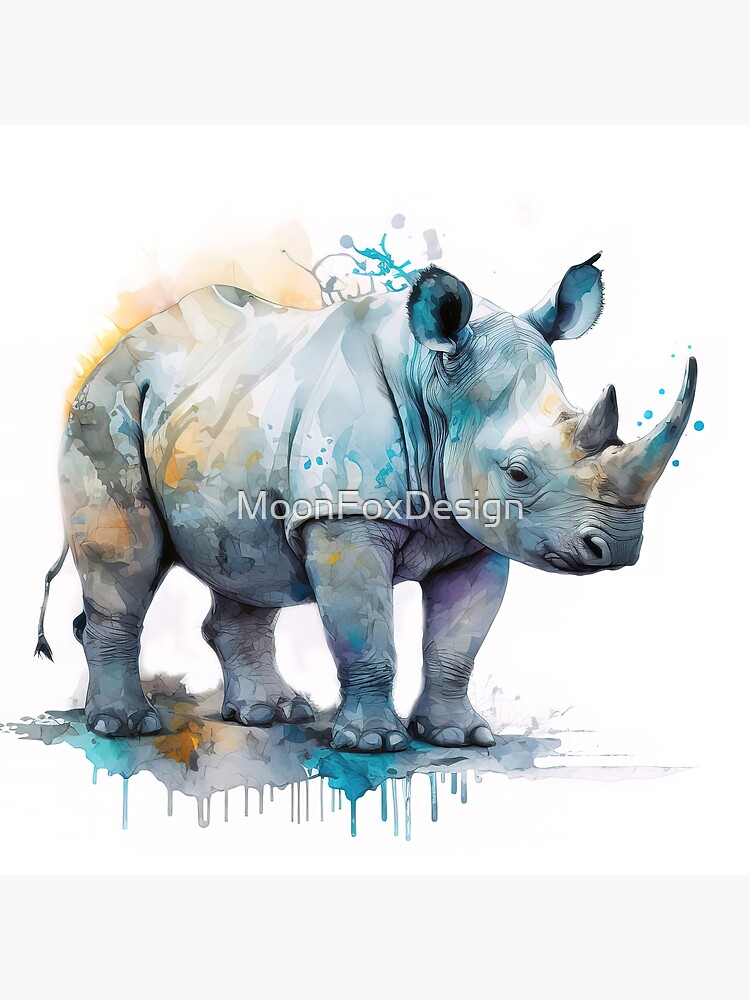This image is a digital watercolor illustration of a life-like rhinoceros, created with a pen and ink style and overlaid with vivid watercolor effects. The rhino is standing with its head to the right and its back leg to the left, showcasing detailed, wrinkled skin shaded intricately with pen and ink. The watercolor glazing enhances the scene with drippy, paint-splattered textures in vibrant hues of blue, yellow, purple, and gray. Some parts of the watercolor appear almost inorganic, as the colors do not blend together seamlessly. The rhinoceros casts a subtle shadow on the plain white background, which has soft off-white strips along the top and bottom edges. A transparent watermark reading "Moon Fox Design" in white text with a drop shadow stretches across the middle of the image. The serene white background intensifies the vibrant paint splatters, giving an impression of blue and yellow paint almost dripping off the rhino, emphasizing its distinctive paint-thrown aesthetic. The ears of the rhinoceros are perked up, adding to the realism and dynamic feel of the piece.